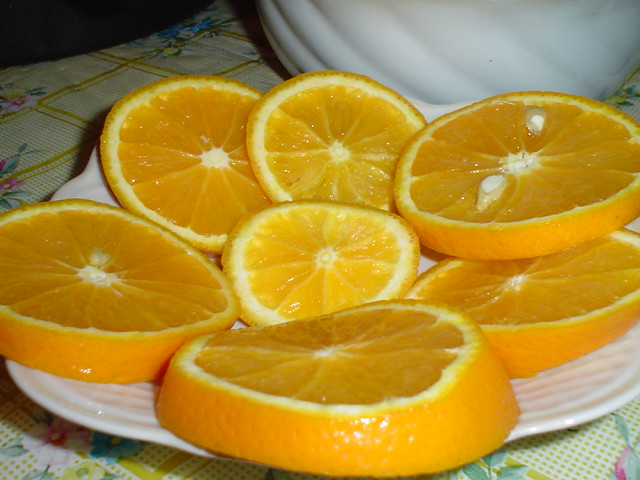This image features seven thin slices of orange arranged on a white plate, with each slice showcasing a dark orange peel and a distinct white circular center. The slices display a radial pattern, with lines extending from the white center out towards the peel. One slice in the middle appears smaller, thinner, and lighter than the rest. Some slices have small seeds attached to the inner pulp. The arrangement slightly overlaps the edge of the plate, creating a casual, natural display. The plate itself sits atop a green tablecloth adorned with yellow squares and floral patterns, adding a vibrant background. Nearby, a white ceramic container with curving lines up its sides complements the setting. A reflection of light glistens on the peel of the slice nearest to the edge, highlighting the texture and freshness of the fruit.